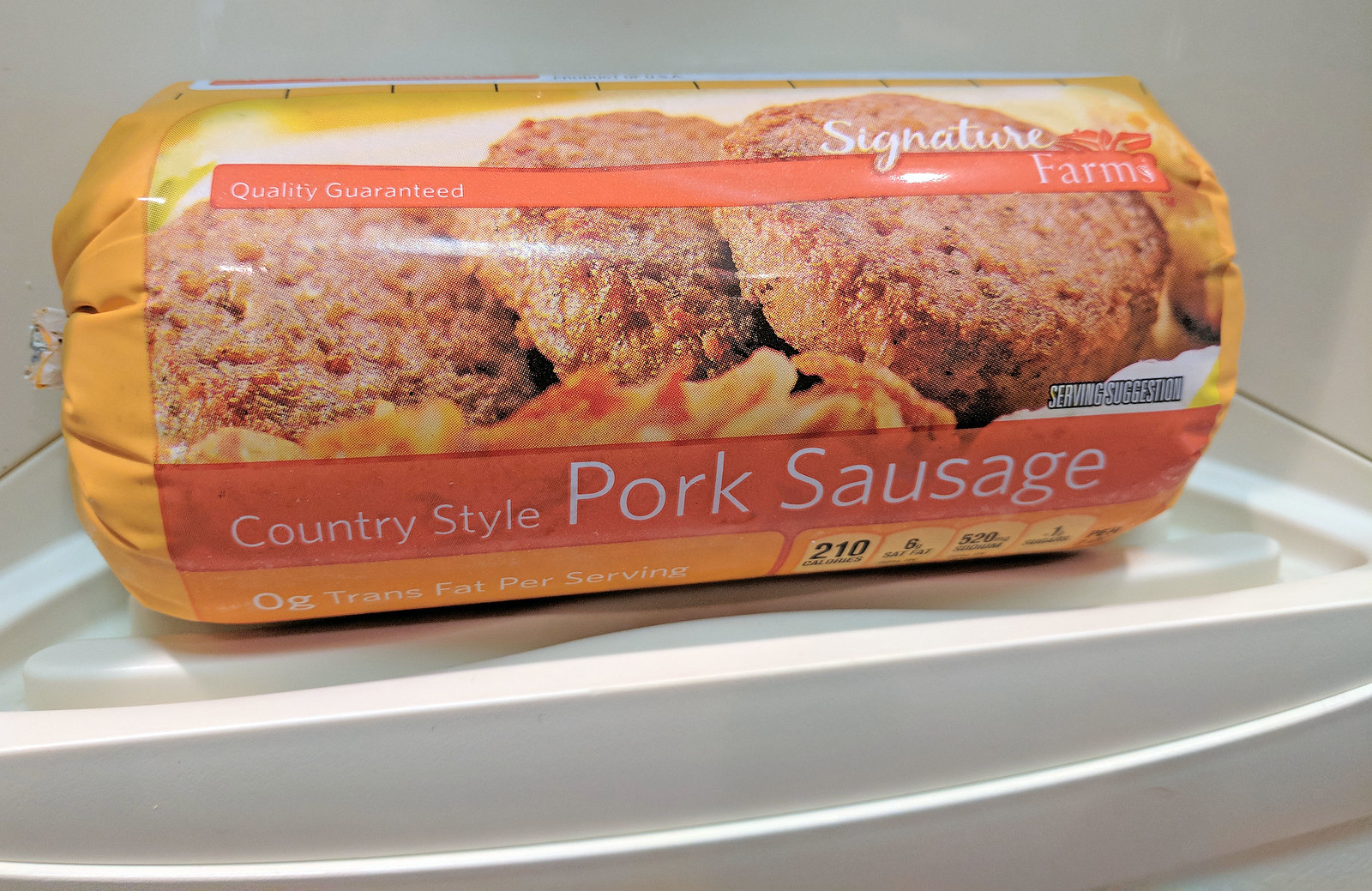This close-up photograph showcases a vibrant and detailed packaging of Signature Farms' Country-Style Pork Sausage, which is frozen and ready for cooking. The cylindrical package is adorned with colorful graphics, prominently featuring an appetizing image of cooked sausages paired with what appears to be French fries. Key information is clearly displayed on the packaging, including the product title, the brand name "Signature Farms," and a quality guarantee. A serving suggestion is present, noting the sausage contains zero grams of trans fat per serving and has 210 calories. The package rests on a triangular white platform, likely within a refrigerator or freezer, although the exact location is ambiguous due to the close-up nature of the photo.